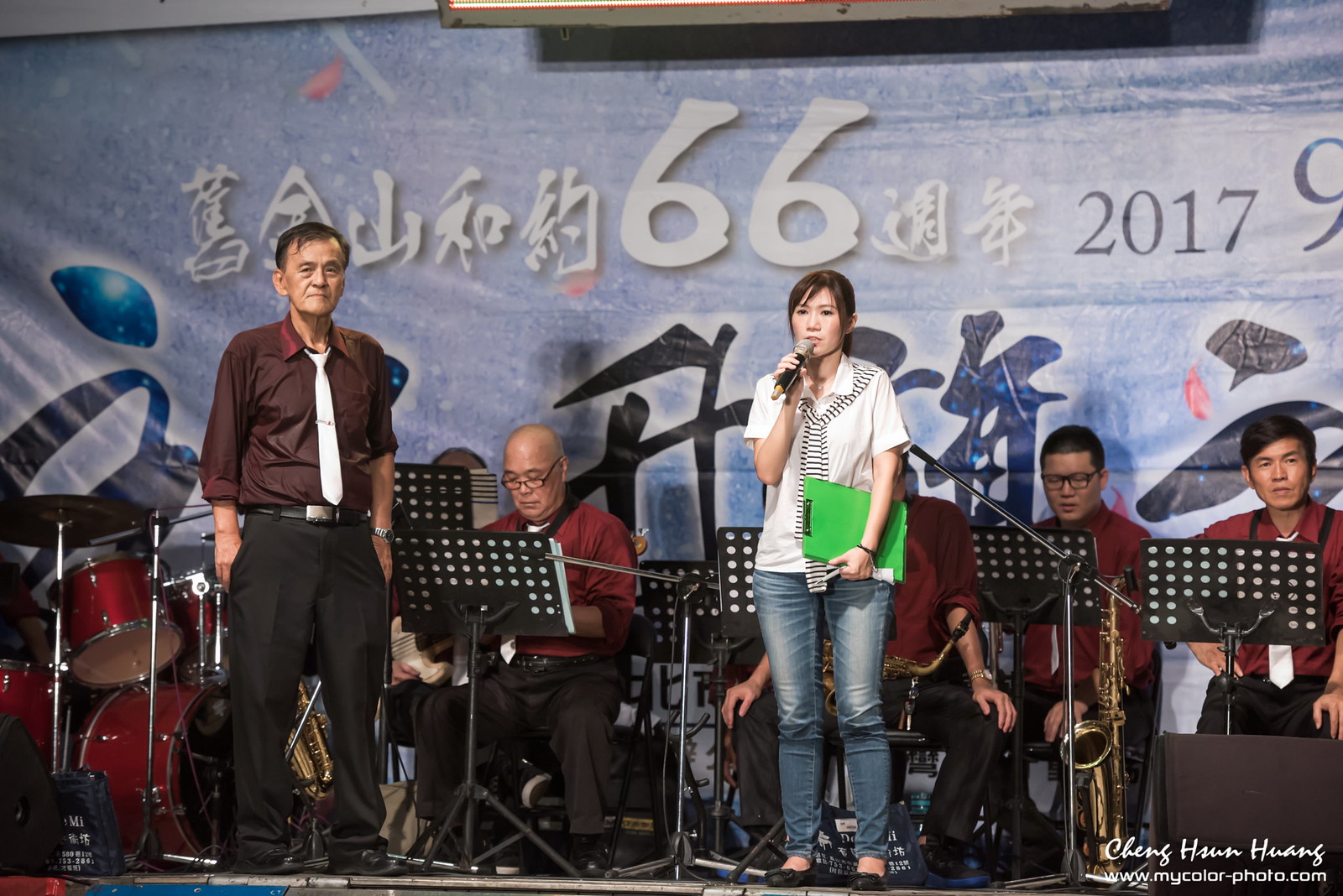The image captures an indoor musical performance setting. In the foreground, a woman stands holding a microphone in her right hand and a green notebook in her left. She is dressed in blue jeans, a white shirt, and a black and white striped scarf. Behind her, several men dressed in maroon shirts are seated, each with musical instruments such as saxophones and brass instruments, and are reading from sheet music placed on stands in front of them. A man in dress pants, a maroon shirt, and a white tie stands nearby with his hands in his pockets. On the far left, there is a burgundy-colored drum set. The back wall features a large banner with Chinese or Japanese characters, a '6-6' symbol in the center, and '2017' to the right. The banner has a light blue background with white and darker blue characters.